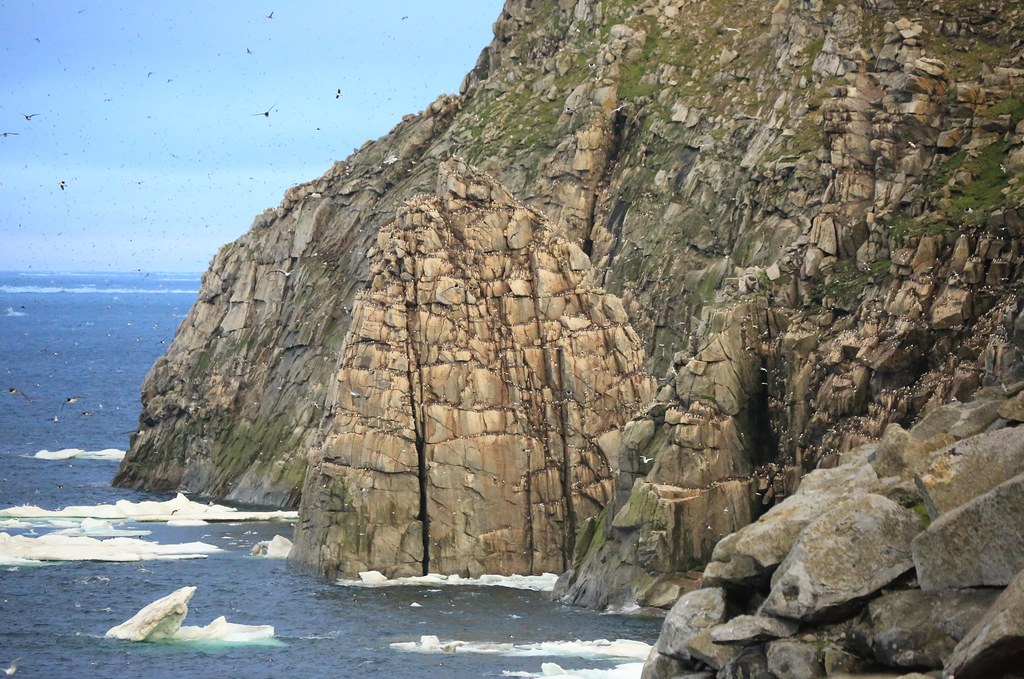In this photograph, a majestic, rugged cliff dominates the scene, extending from the center to the right side of the image. The cliff is predominantly brown, adorned with patches of green that suggest the presence of grass or small shrubs. The surface of the cliff is rich with cracks and intricate patterns, adding to its rugged charm. Scattered across the cliffside are small white speckles that resemble birds.

To the left side of the photograph, the upper portion reveals a light blue sky filled with numerous black specks, which are birds in flight. These birds are also seen closer to the dark blue ocean below, where patches of ice float on the choppy water, highlighting the cold environment. The ocean spans from the center to the front of the image, with medium to small ice chunks scattered across its surface. The striking composition of the blue sky, the icy ocean, and the imposing brown cliff with green accents creates a vivid and detailed portrayal of this frigid coastal landscape.